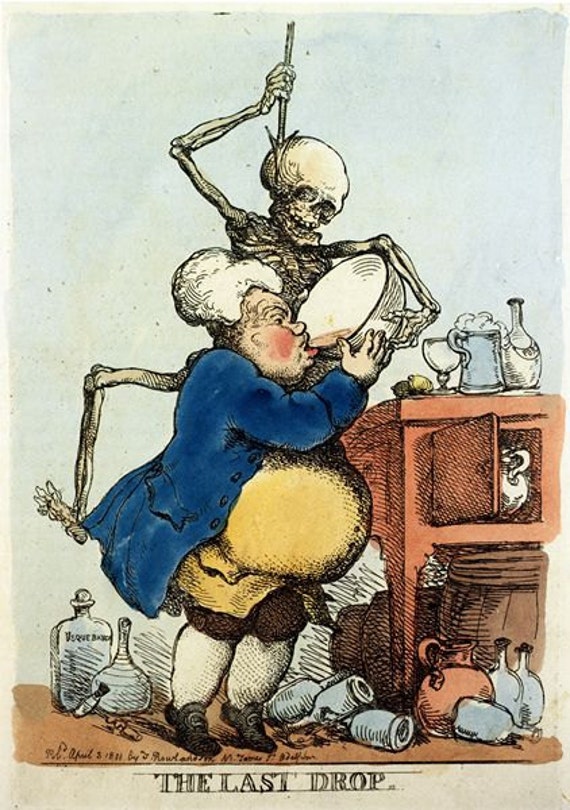The image is a vertically rectangular multi-colored print piece with a thin border on the top, bottom, and sides, though the bottom border is slightly thicker and features the black text "The Last Drop." In the scene, a man dressed in 1770s attire is depicted with black shoes, white stockings, black knee-length pants, a yellow shirt stretched over a massive belly, a blue jacket, and a white wig. He is drinking from a large cream-colored bowl containing a light brown liquid. Behind him stands a dancing skeleton with a spear pointed ominously at the man's head. At the man's feet are several empty bottles, and a counter to his right holds additional bottles, a beer mug, and a brown chest with an open window door. On top of the chest are various vessels, including a glass cup, a light blue mug, and a white beaker, suggesting he has indulged in their contents.